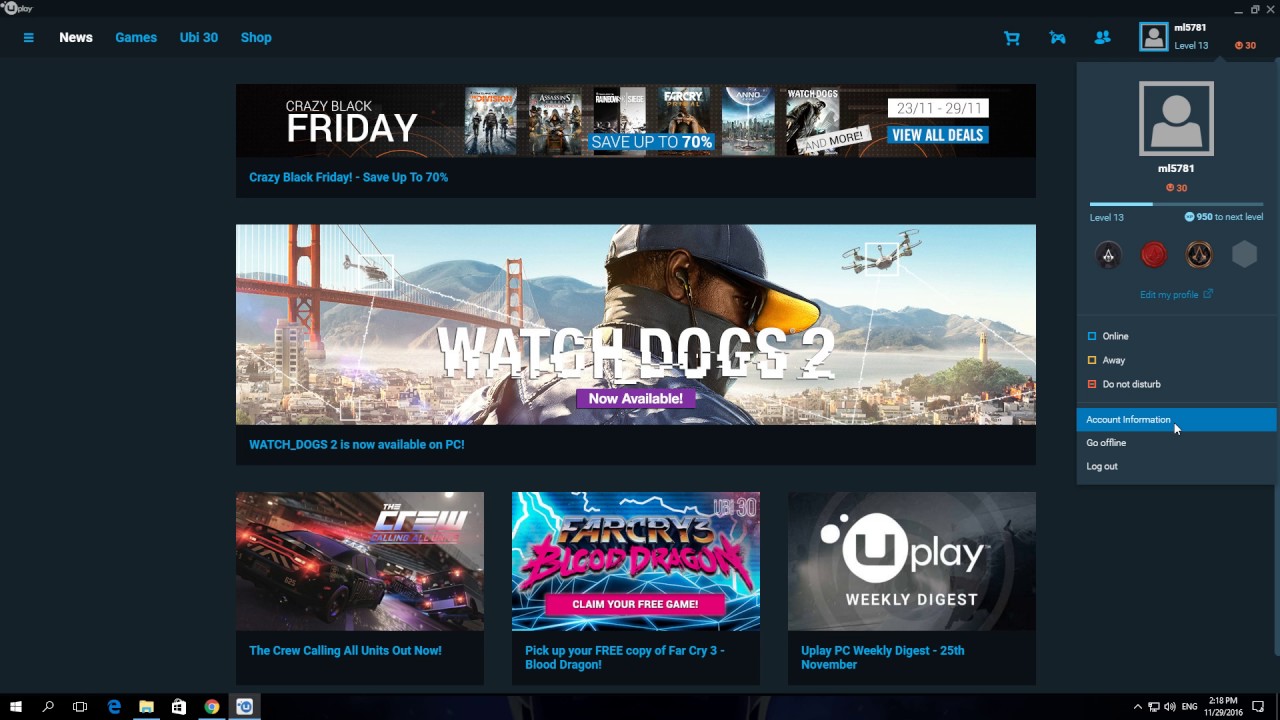### Detailed Caption of the Image

The image is a left-to-right horizontal screenshot that resembles a computer screen with a primarily black background, appearing somewhat dull. The bottom of the screen features a darker jet-black strip, creating a contrast that makes the middle area look lighter.

In the upper left-hand corner, a play icon and three horizontal blue lines are visible. The word "News" is prominently highlighted in white, while adjacent tabs labeled "Games," "UBL 30," and "Shop" are displayed in blue.

On the upper right corner, the familiar minimize, maximize, and close buttons (X) are present. Below this, there is a row that includes a shopping cart icon, followed by smaller icons resembling Nintendo controllers, and a profile picture symbol. This profile box shows the username "MLS 5781" or "ML 5781," with an indication of level 13 and some numerical value, possibly "30."

Prominently, a message reads "Set Crazy Black Friday," accompanied by various game cover images with the text "Save up to 70% and more" and the promotional dates "23-11 to 29-11." A "View All Deals" button is included. A section advertises "Watch Dogs 2 Now Available," featuring an image of the Golden Gate Bridge, a person, and helicopters. There's a tagline noting its availability on PC.

Another game called "The Crew: Calling All Units" is highlighted, suggesting vigilance for free offers such as "Far Cry 3 Blood Dragon." The date "25th of November" is mentioned, associated with the "Uplay Weekly Digest."

Icons for determining user status ("Online," "Away," "Do Not Disturb"), account options such as "Go Offline" and "Log Out" are displayed near the bottom.

Finally, the bottom of the screen includes standard icons found on a computer taskbar: Internet Explorer, Chrome, time, and date, displayed in the bottom-right corner.